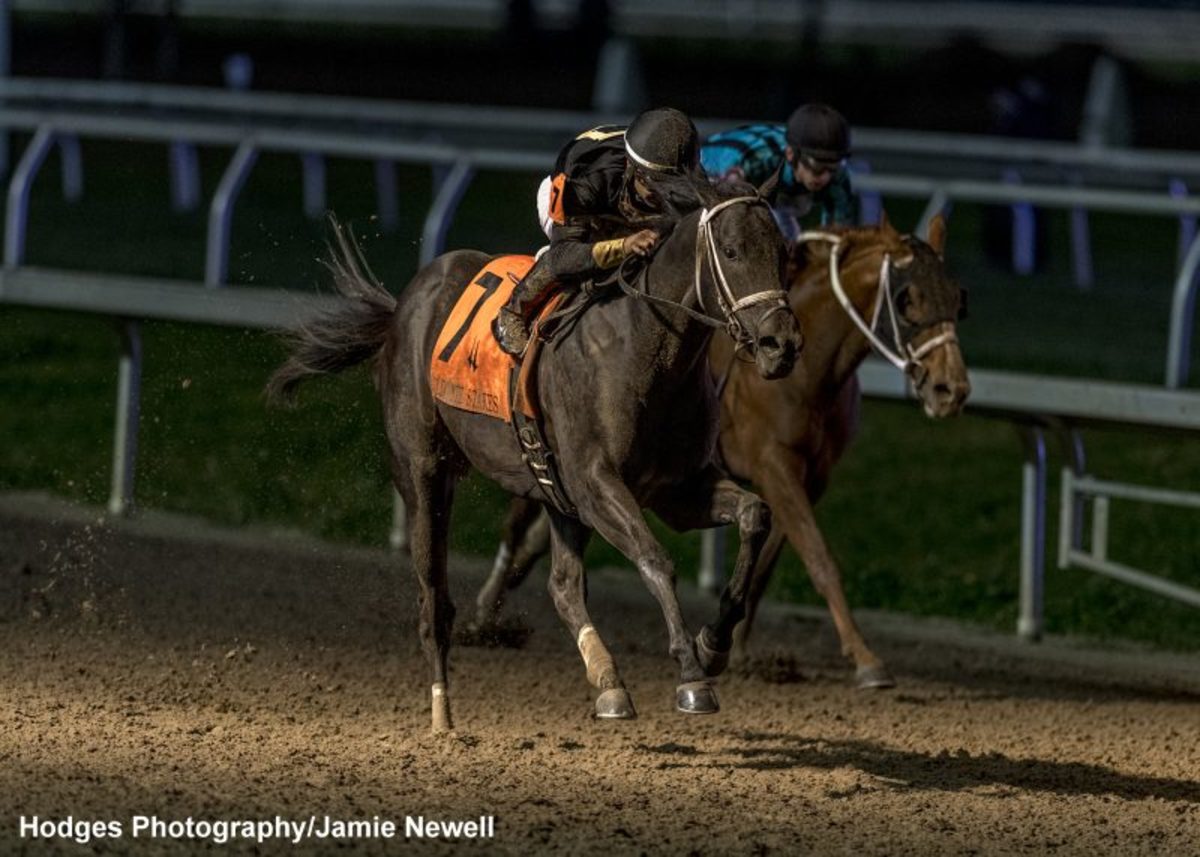This professionally captured, high-resolution photograph by Hodges Photography / Jamie Newell depicts an intense moment in a horse race. The two racehorses, racing neck and neck on a dirt track, vividly showcase their jockeys' competitive spirit. The jockey on the dark grayish-brown horse, which has the number 7 on its blanket, is dressed in a black cap, black shirt, white pants, and brown boots. This jockey is crouched low, poised for victory. The second jockey, riding a slightly lighter brown horse on the inside rail, wears a black helmet and a blue shirt with black stripes, also leaning forward in a determined stance. Both horses appear incredibly close together, emphasizing the thrilling nature of the race. The background reveals a section of the racetrack's railing and a hint of grass, adding context to the setting. The bottom left corner of the image is marked with "Hodges Photography / Jamie Newell," crediting the creators of this dynamic and detailed scene.